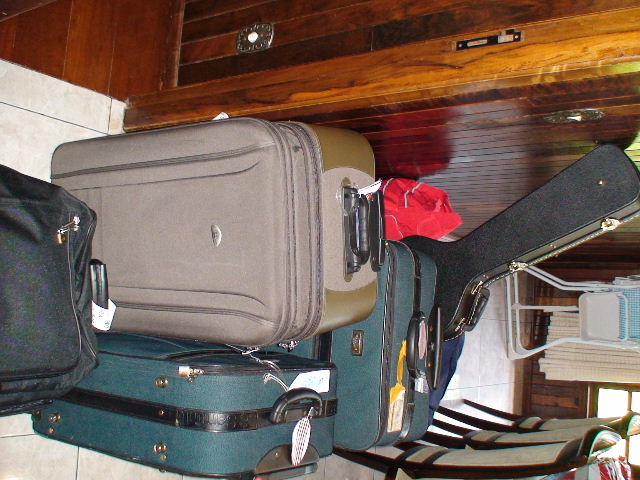The digital photo, taken indoors and currently displayed sideways, captures an arrangement of several suitcases leaning against a doorway. Prominently, there is a black hard case for a guitar, suggestive of an acoustic type. The floor, which should be viewed as the bottom but appears at the top due to the photo's orientation, consists of a dark wood planked surface, while the lower part of the image shows a white tiled floor with gray grout.

The variety of luggage includes a brown, a gray/silver suitcase, two turquoise (or dark cyan) suitcases with black handles, a small black suitcase, and a red, white, and gray bag that may be perched on one of the chairs. The scene suggests preparation for travel, indicating someone might be coming or going. 

In the background, there are dining room chairs with black wood and gray cushioning and a foldable chair. These are set against walls made from wood panels of varying shades, primarily a dark red wood. Windows with curtains further frame the background, contributing to the sense that this could be within an RV or camper van.